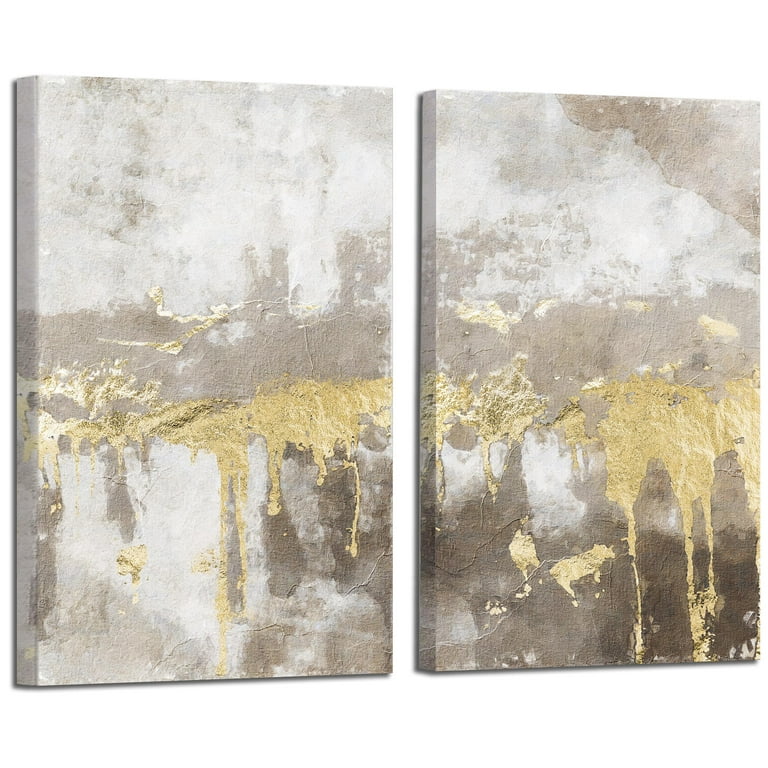The image showcases two vertical rectangular paintings hung side by side, resembling two canvases each with distinct yet complementary abstract designs. The canvas on the right features a dominant brown hue at the top corner, fragmented by white speckles that disperse across the surface. A splash of gray paint blends into patches of white, contrasted by streaks of yellow paint that drip downward, culminating in a vibrant brown speckled effect.

The left canvas, in harmony with the right, exhibits a significant presence of white paint stretching from the left to the right, interspersed with patches of gray. The yellow paint, which seems to mimic dripping or cracking plaster, descends subtly into the lower sections of the painting. The background transitions into dark gray at the bottom, with the gray becoming increasingly prominent toward the bottom right corner.

Both canvases, characterized by thick, splotched, and heavily brushed paint, form an abstract composition that bears elements of a weathered stone wall with a marble-like pattern, showcasing an interplay of white, gray, yellow, and brown tones. The paintings, framed and textured, do not depict identifiable objects but rather evoke feelings through their bold use of colors and organic patterns.